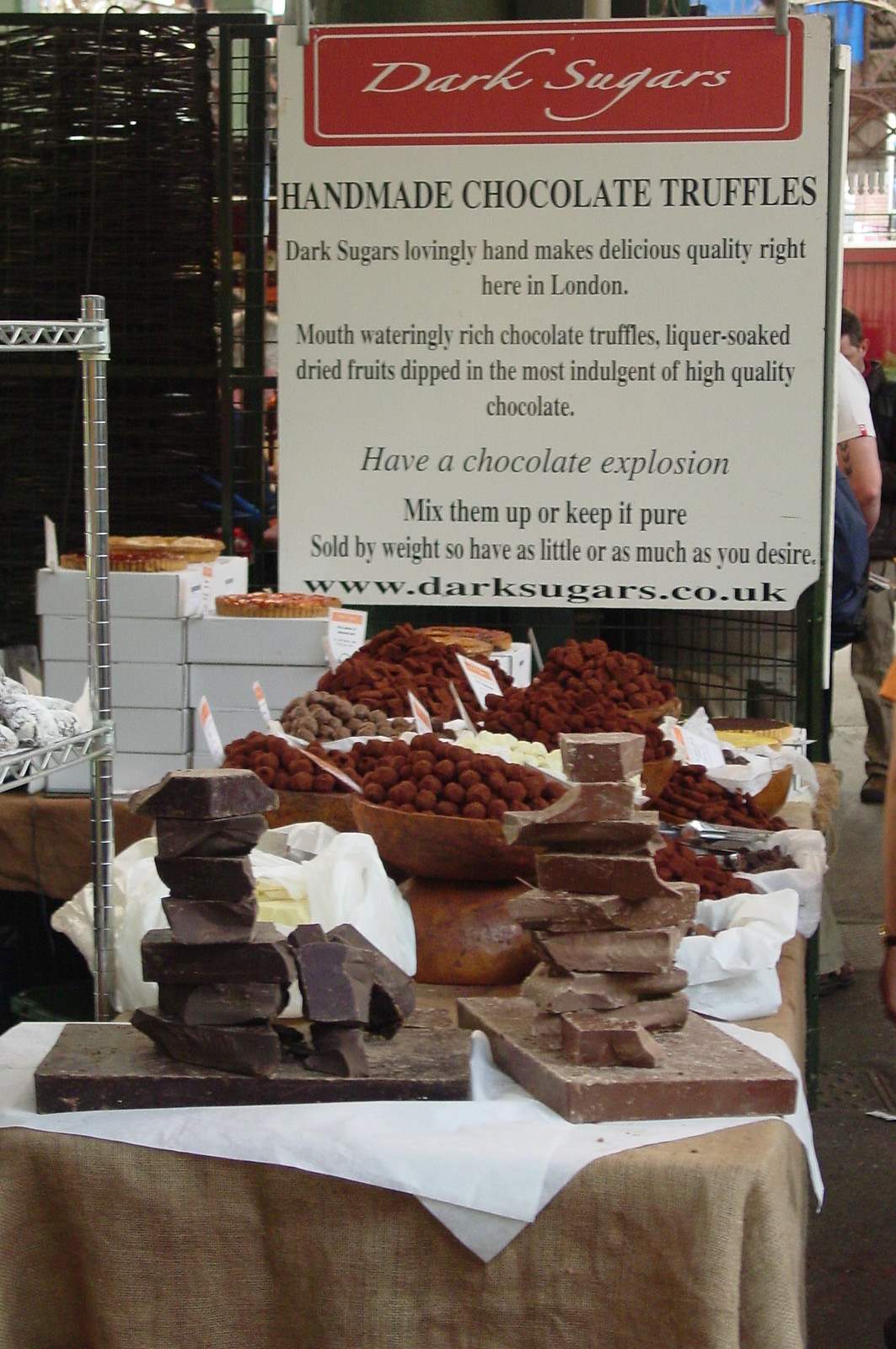In the image, there's a detailed setup at a booth featuring an enticing display of chocolates. Dominating the table is a long rectangular arrangement showcasing an assortment of large chocolate blocks, including dark, milk, and white varieties, some of which are stacked on top of each other resembling cutting boards. Behind these impressive slabs are two rows of four large brown bowls, each filled with small, pebble-shaped handmade chocolate truffles. The truffles are various shades of brown, hinting at the rich and diverse flavors.

Above the delectable display is a prominent sign. The sign has a bold red rectangle at the top with the words "Dark Sugars" written in elegant white script, accentuated by a thin white outline. Beneath this, in clear black ink, it states "Handmade Chocolate Truffles." The detailed description extols the craftsmanship and quality of the truffles, highlighting that they are lovingly handmade right in London. It mentions features like mouth-watering richness, liqueur-soaked dried fruits, and the use of the most indulgent high-quality chocolate, encouraging customers to experience a "chocolate explosion" either by mixing the varieties or savoring them individually. It also notes that the chocolates are sold by weight, allowing for customizable quantities. The sign closes with the company’s website, www.darksugars.co.uk, making it easy for enthusiasts to find more information online.